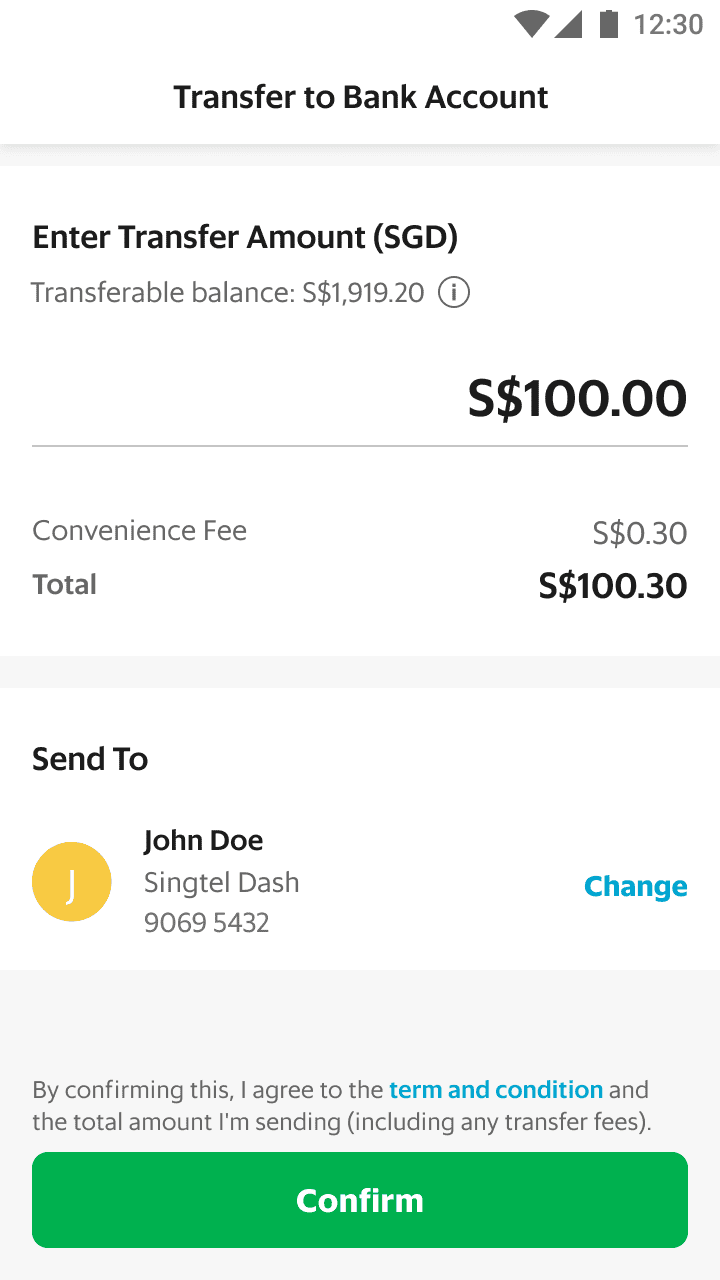The top of the screenshot displays a Wi-Fi signal icon, a battery icon, and the current time, 12:30 PM. Below, there is a section labeled "Transfer to Bank Account." A gray area beneath that prompts the user to "Enter Transfer Amount (SGD)." The transferable balance is shown as S$1,919.20, accompanied by an information icon (a circle with a lowercase 'i' inside). 

The user has entered an amount of S$100.00 in bold black text. A gray line separates this amount from the "S$0.30 Convenience Fee," leading to a total of "S$100.30." 

Further down, the caption states "Send to," followed by a yellow oval containing the initial 'J' and the name "John Doe." It also includes the phone number format "Singtel - 9069 5432." On the right side of this section is a blue hyperlink labeled "Change."